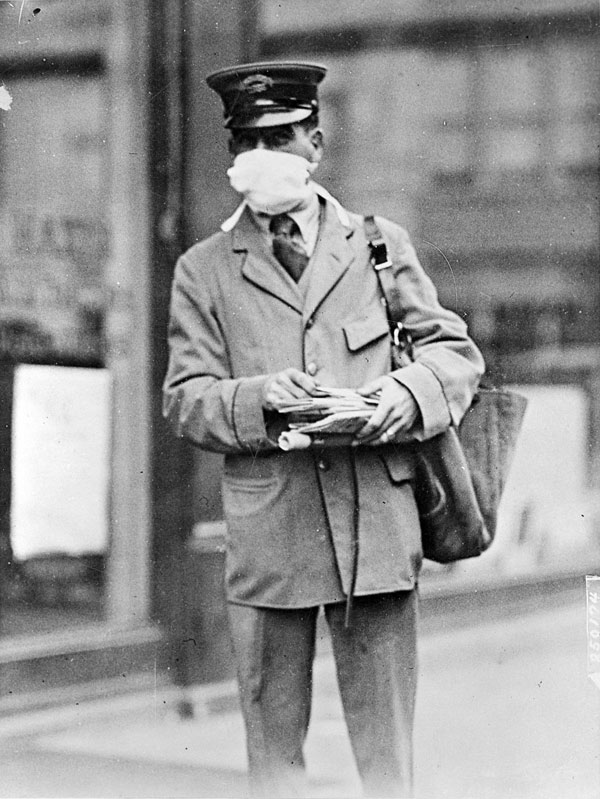A black and white, vertically rectangular photograph captures a historical scene featuring a uniformed mailman standing outdoors on a street during the day. This image, likely from the 1920s or 1930s, shows the mail carrier dressed in a formal suit and tie, topped with a distinctive police-like hat, and a white mask obscuring part of his face. A satchel hangs across his left shoulder, and he clutches a bundle of envelopes in his hands. The background includes out-of-focus buildings and a glass storefront, adding an urban context to the scene. The lighting is natural, with sections of the lower right corner appearing washed out, possibly due to overexposure. The mailman is positioned centrally in the frame, his body facing forward while he looks off to the right, giving a candid feel to the image. The photograph has no borders or text, emphasizing the grayscale palette of black, white, and gray tones.